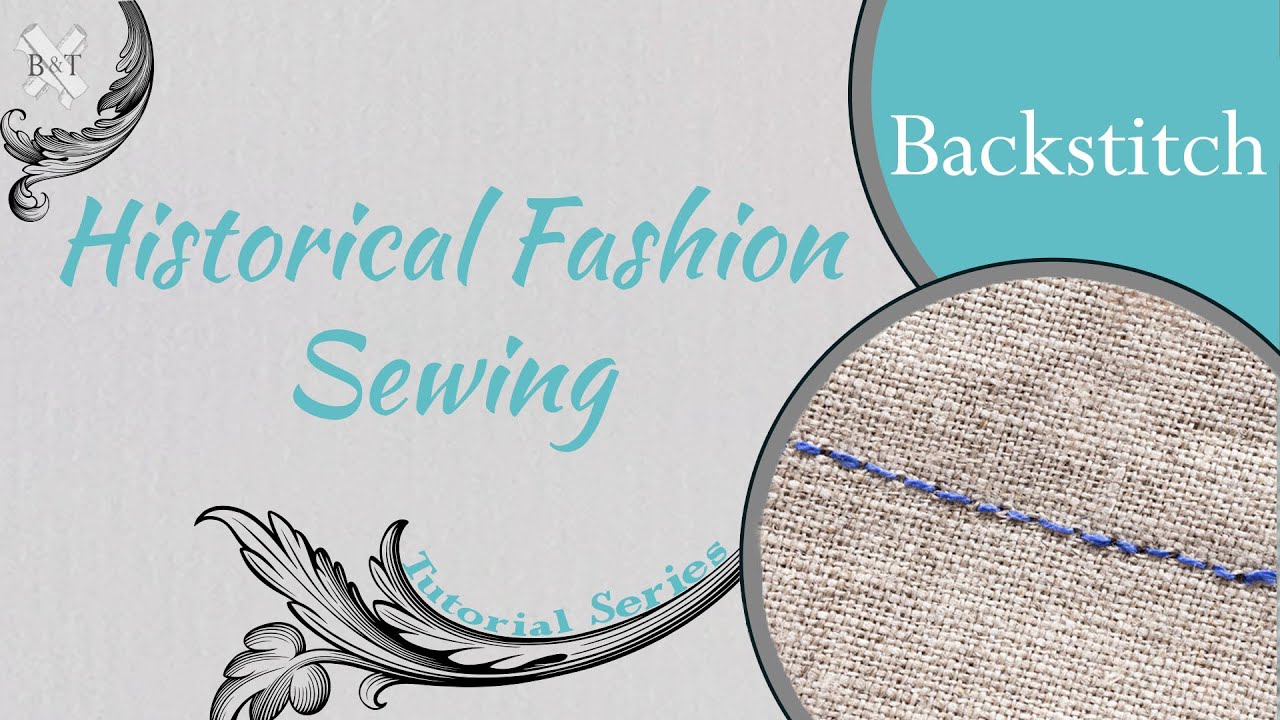The image is a horizontal rectangle with a predominantly gray background. At the top center, the teal-colored text reads "Historical Fashion," followed by "Sewing" beneath it. Positioned in the upper left corner are two white Xs with the initials "B&T" in black, surrounded by a decorative, grayish half-moon emblem. In the bottom section of the image, a large brown circle with blue backstitching runs horizontally across its diameter. This circle features intricate, plant-like patterns extending about three inches from its side. In the same teal color, the text "Tutorial Series" is displayed at a slant above the circle. To the upper right of this circle is another decorative swirl in gray, which loops down and meets the circle. Inside this area, the circle's interior turns teal, with the word "Backstitch" written in white letters.